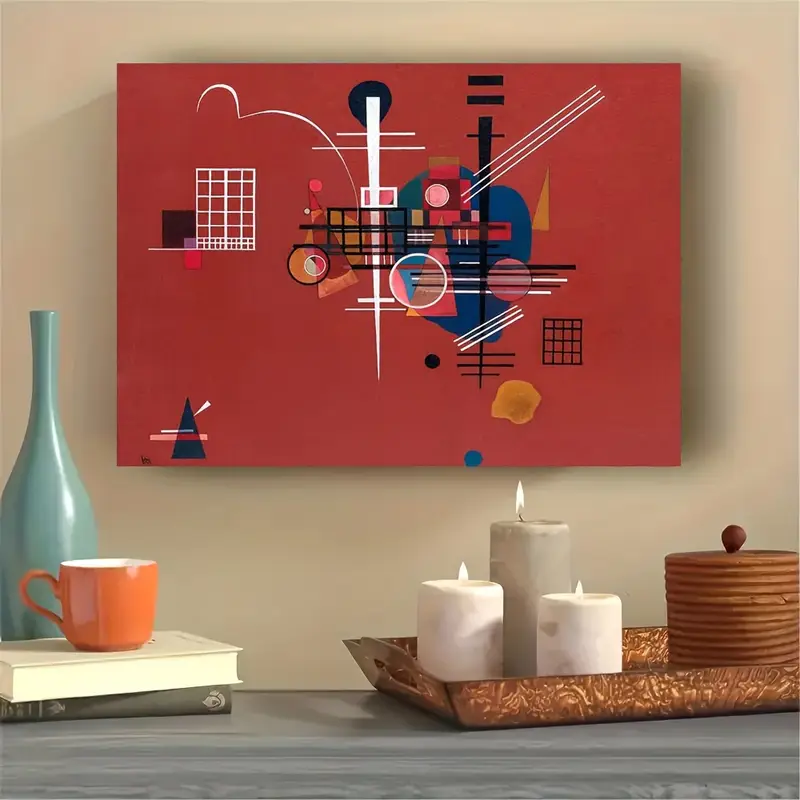The image depicts a detailed interior scene featuring a modern decor arrangement on a gray wooden table against a beige wall. Dominating the background is an abstract, digitally rendered artwork with a striking red backdrop, embellished with various geometric shapes and symbols in colors such as dark blue, white, pink, orange, and black. Among these are a prominent white needle extending from top to bottom and a triangle with horizontal lines in the lower left.

In the foreground, the right side of the gray table showcases a brown and beige tray holding three lit candles: two shorter white cylindrical candles in the front and a taller gray candle behind them. Alongside the candles, the tray also contains a brown jar with a rounded knob on the lid. To the left, there are two stacked books, one gray and the other white, upon which rests an orange coffee cup with a white interior. Behind the stack of books, there is a slender, long-necked blue vase with a narrow opening, adding a touch of elegance to the setting.

This vivid composition blends colorful art and muted decor elements, creating a cohesive and aesthetically pleasing scene.